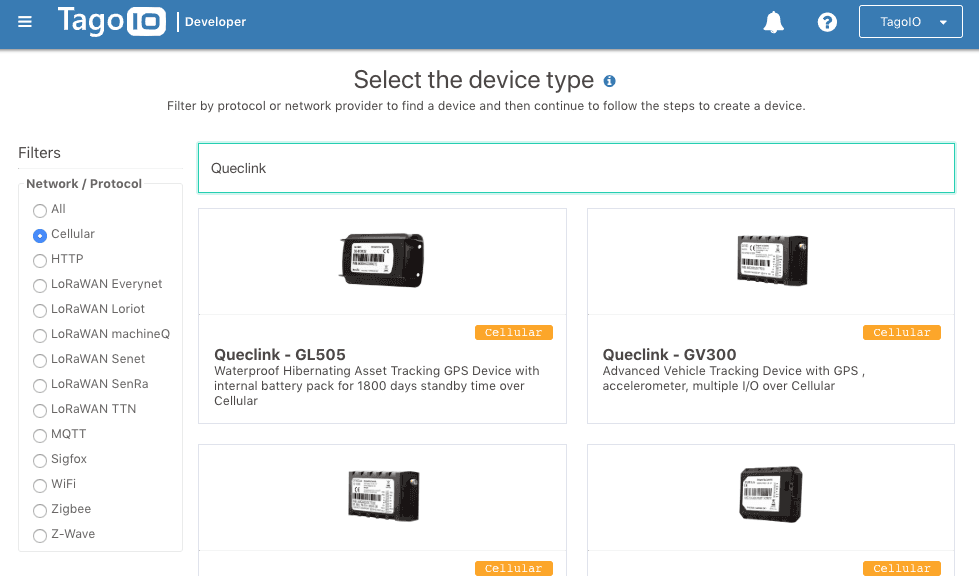This screenshot captures a company's webpage with a comprehensive and organized layout, prominently showcasing their services and options for developers. 

At the very top of the page, on a blue bar, there is a simplified navigation icon represented by three horizontal lines. The company's name, "TagoIO/Developer," is displayed in white text, except for "IO" which is emphasized in blue within a white box, creating a visually striking and clear identifier.

The blue bar also hosts icons such as an alarm and a question mark, likely serving as quick-access tools or help options. Additionally, there is a scrolling box, though its purpose is not described in detail.

The main content of the page is set against a white background and features a selection interface for device types. It includes options to filter by protocol and network provider, with a vertical sidebar offering additional filtering criteria such as "filters," "network," and "protocol." "Cellular" is the currently selected protocol, along with "HTTP." The interface allows the user to manage and view numerous devices, as indicated by a list of approximately 20 different computer names.

The central section of the page highlights four different types of devices, specifically Q-Liq NIC, each offering unique functionalities. Detailed descriptions for each device are provided, including attributes like "waterproof," and "hibernating asset tracking," alongside a "GPS device with an internal battery pack offering up to 1800 days of standby time over cellular."

This clean, detail-oriented design facilitates easy navigation and thorough exploration of the wide array of device options available to developers.